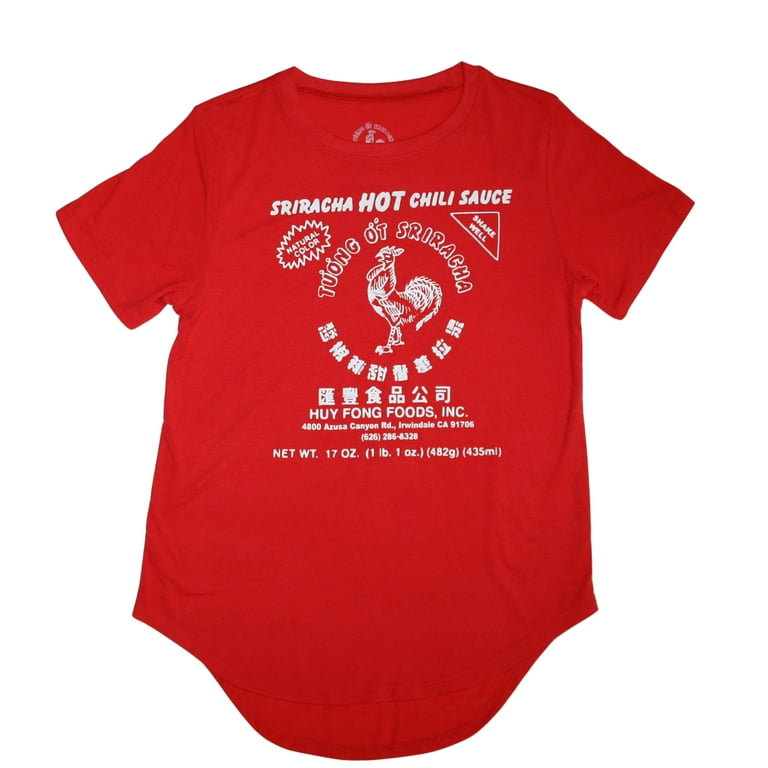This image showcases a bright red, short-sleeved t-shirt against a white background, designed to mimic a bottle of Sriracha hot chili sauce. Dominating the center of the shirt is a detailed white print of the iconic Sriracha label. At the top, it reads "Sriracha Hot Chili Sauce" with a circular "Natural Color" bubble on the left and "Shake Well" with a small clockwise circle on the right. The print prominently features the well-known rooster logo positioned centrally with the words "Tuong Ot Sriracha" above it. Underneath the rooster, a mix of Vietnamese and Chinese characters is visible, followed by "Huy Fong Foods, Inc.," along with the company’s address at 4800 Azusa Canyon Road, Irwindale, CA 91706, and phone number 626-285-6326. The measurement details at the bottom state the weight as "Net Wt 17 oz (482 grams, 435 milliliters)." The shirt's design faithfully replicates the look of a Sriracha bottle, employing only red and white colors, and includes every distinctive label element down to the metric measurements.